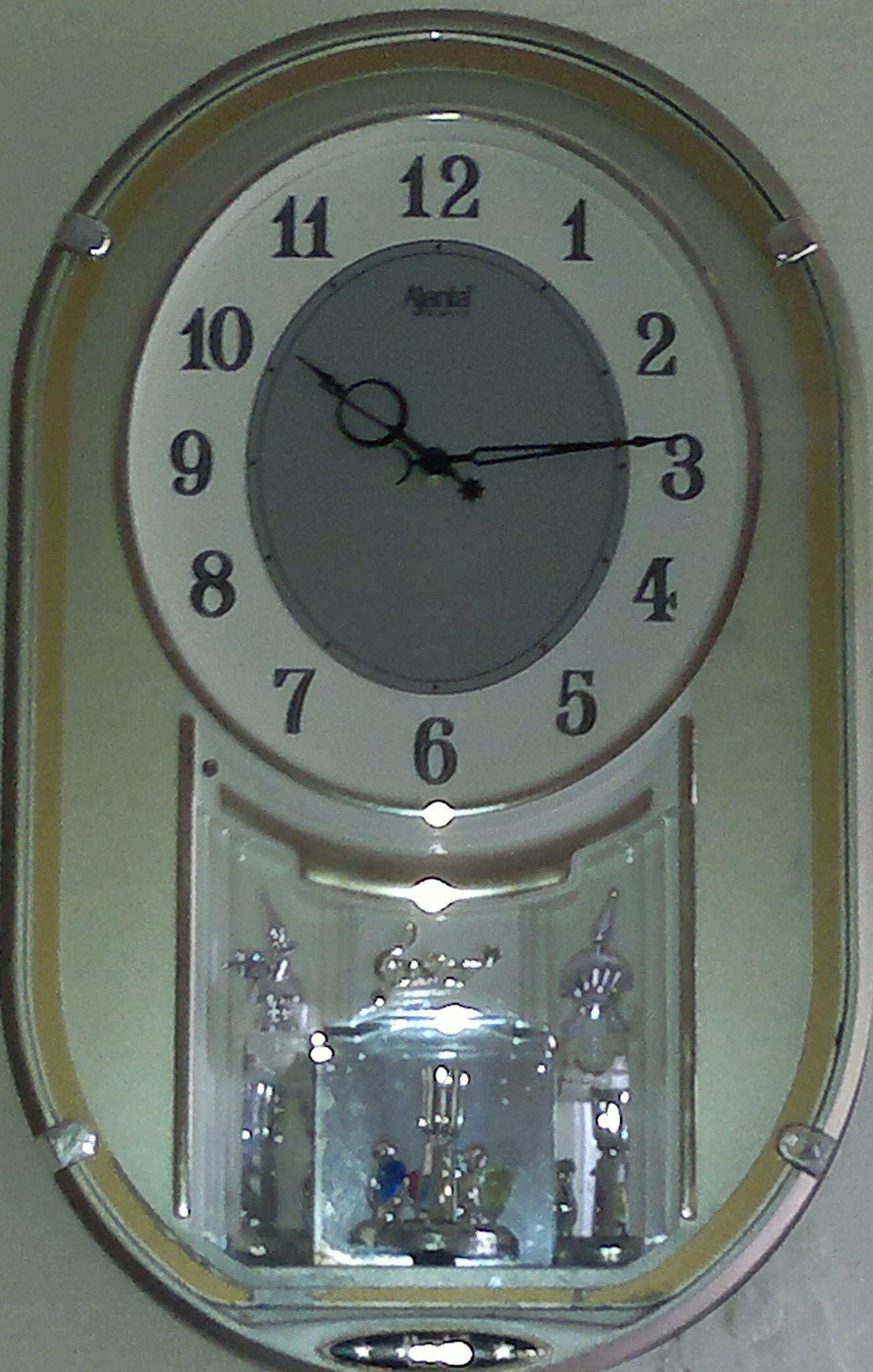This is an image of a unique, oval-shaped wall clock hanging on an off-white or beige wall. The clock consists of two main sections: a circular clock face at the top and a trophy-like display case below it. The clock face features black numbers and black hands, with a white outer ring and a gray center. The hour hand has a distinctive circle at its tip, and the time shown is 10:14. The entire clock is encased in a thin, silver metal frame with metal brackets securing the front glass panel at each corner. Below the clock face, a display case houses small, metallic, silver-colored figurines, reminiscent of trophy-like items or dancing figures. Some of these figurines include characters wearing colorful outfits, such as a green dress and a blue jacket, adding a touch of charm to the otherwise sleek, metallic aesthetic.